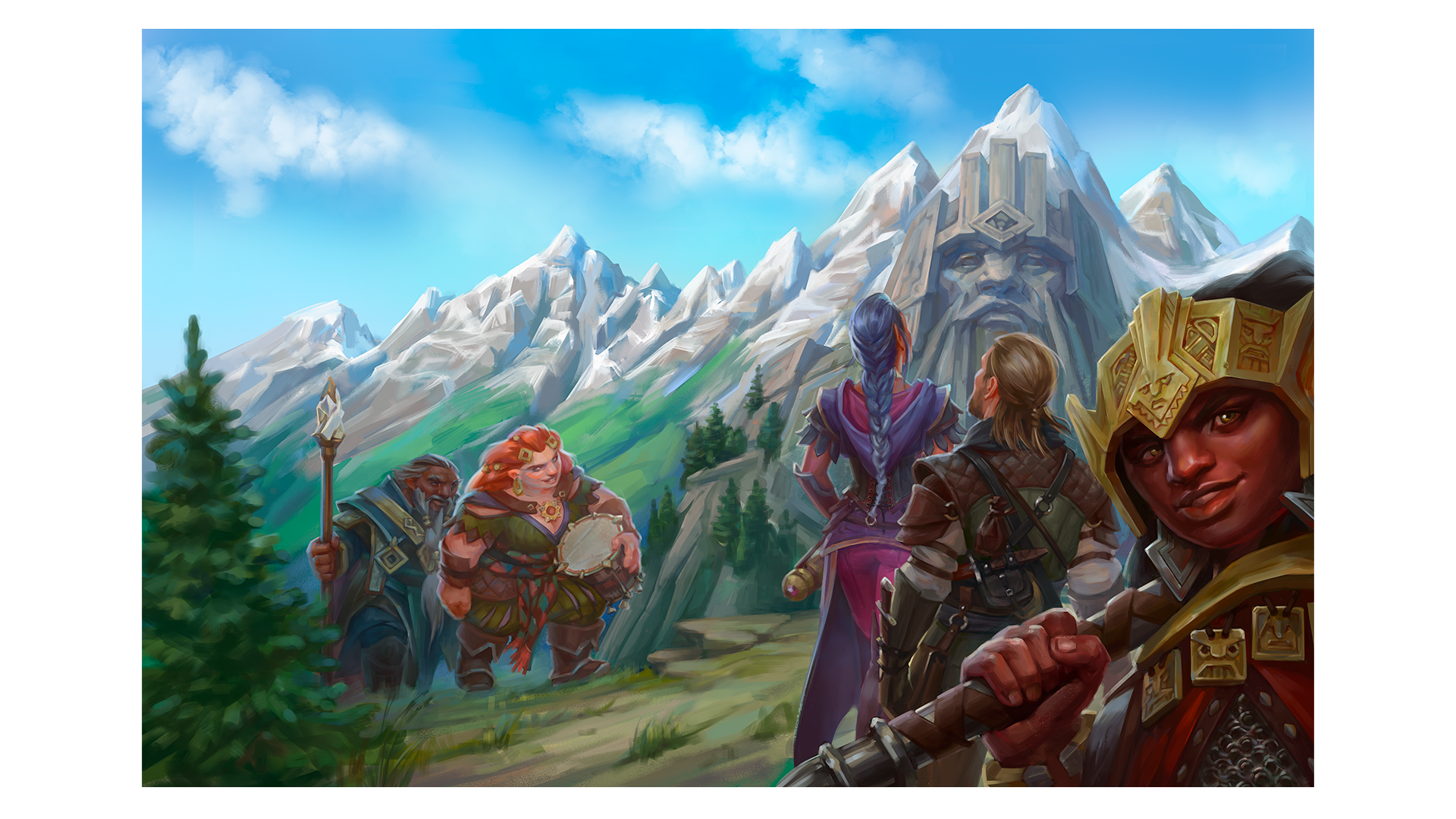The image presents a high fantasy setting characterized by a stunning, digitally created landscape. A clear blue sky dotted with white clouds serves as the backdrop, above snow-capped grey mountains that cascade into lush green valleys. In the left lower corner, a prominent pine tree stands, anchoring the scene. The picture features five characters, each with unique attire and accessories that hint at their roles and backgrounds. Beginning in the bottom right corner, a dwarf with a helmet and a sword slung over his shoulder gazes directly at the viewer. Above him, two individuals are positioned: one in a green shirt and pants, holding a torch, and another with a brown robe-like outfit, beating a drum. These two figures appear to be journeying across the mountainside. On the right, two more characters stand with their backs turned, facing a grand statue carved into the mountain rock, resembling a regal figure. One of these figures wears a purple dress and has grey braided hair, while the other is clad in armor. The scene is awash with rich colors: blues, greens, reds, purples, goldish yellow, and whites, enhancing the vibrant, fantastical atmosphere of the artwork.